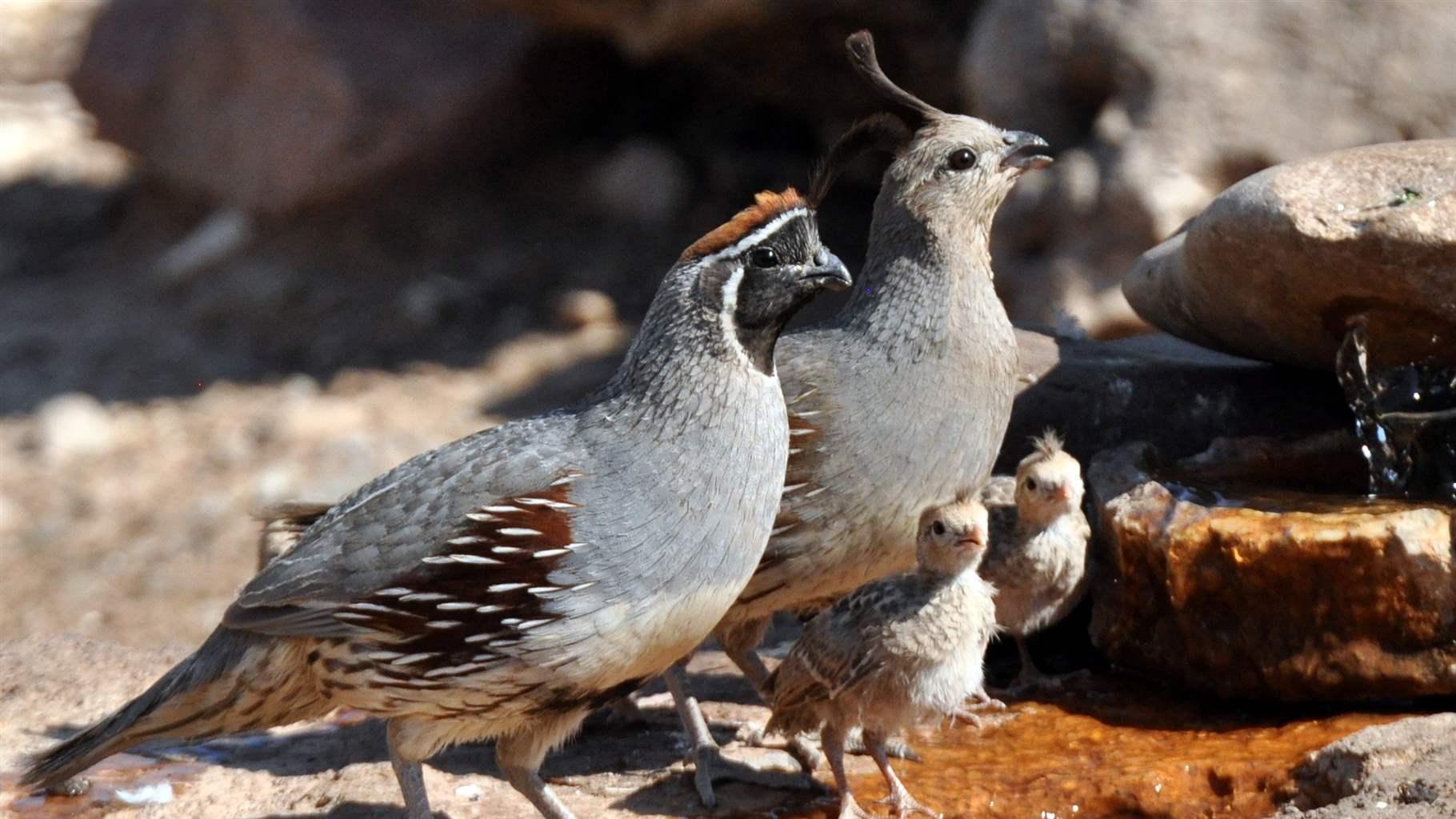Under the bright daytime sun, a close-up image captures a family of four birds perched on the gray rocks of a picturesque, water-splashed rock quarry. The scene is serene and detailed, with two adult birds and two baby birds. One adult bird has a striking black face with white surrounding its head and neck, complemented by a reddish-brown mane and similarly hued wings. The other adult bird features a distinctive gray plumage with a tuft of brown and white feathers on its head. The two fluffy baby birds in front of them are predominantly brown with speckles of white, sporting tufts of fur on their heads and webbed feet. The background showcases large gray rocks and a gentle flow of water, contributing to the natural, tranquil setting.